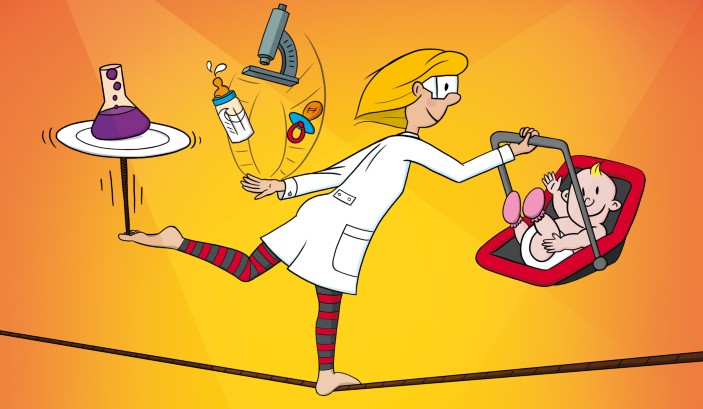This cartoon-style drawing illustrates a woman, likely a mother and a professional scientist, precariously balancing her demanding roles. She stands barefoot on a tightrope with one foot, her left leg extended backward to support a spinning plate on a stick. On the plate is a lab beaker filled with a liquid suspension. The woman, with short blonde hair, wears a white lab coat and safety goggles, emphasizing her scientific profession. Her right arm is extended forward, holding a baby in a car seat, while her left arm, stretched backward, juggles a bottle, baby bottle of milk, a pacifier, and a microscope. The background is a striking yellow, highlighting the chaotic yet comedic essence of trying to balance professional and personal life. She also sports striped leggings, humorously suggesting she might still be in her pajamas, further underscoring the daily circus of her multitasking challenges.